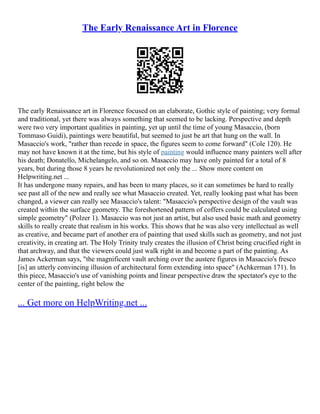The image depicts a dense, text-heavy article on a pure white background. At the top of the image, there's a title in bright blue, underlined text that reads "The Early Renaissance Art in Florence," suggesting it's likely a screenshot from a computer. Below the title is a prominent black QR code. The article consists of two densely packed paragraphs in black text, elaborating on the characteristics and evolution of early Renaissance art in Florence, including notable figures like Donatello and Michelangelo. It discusses how artists such as young Masaccio, also known as Tommaso di Ser Giovanni di Simone, used geometry and perspective to revolutionize the art form, creating an illusion of depth. There is a specific mention of the "Holy Trinity" and a quote by James N. Ackerman highlighting Masaccio's use of vanishing points and linear perspective to create an illusion of architectural form. Towards the bottom of the image, there is another blue underlined hyperlink text that reads "Get more on helpwriting.net."